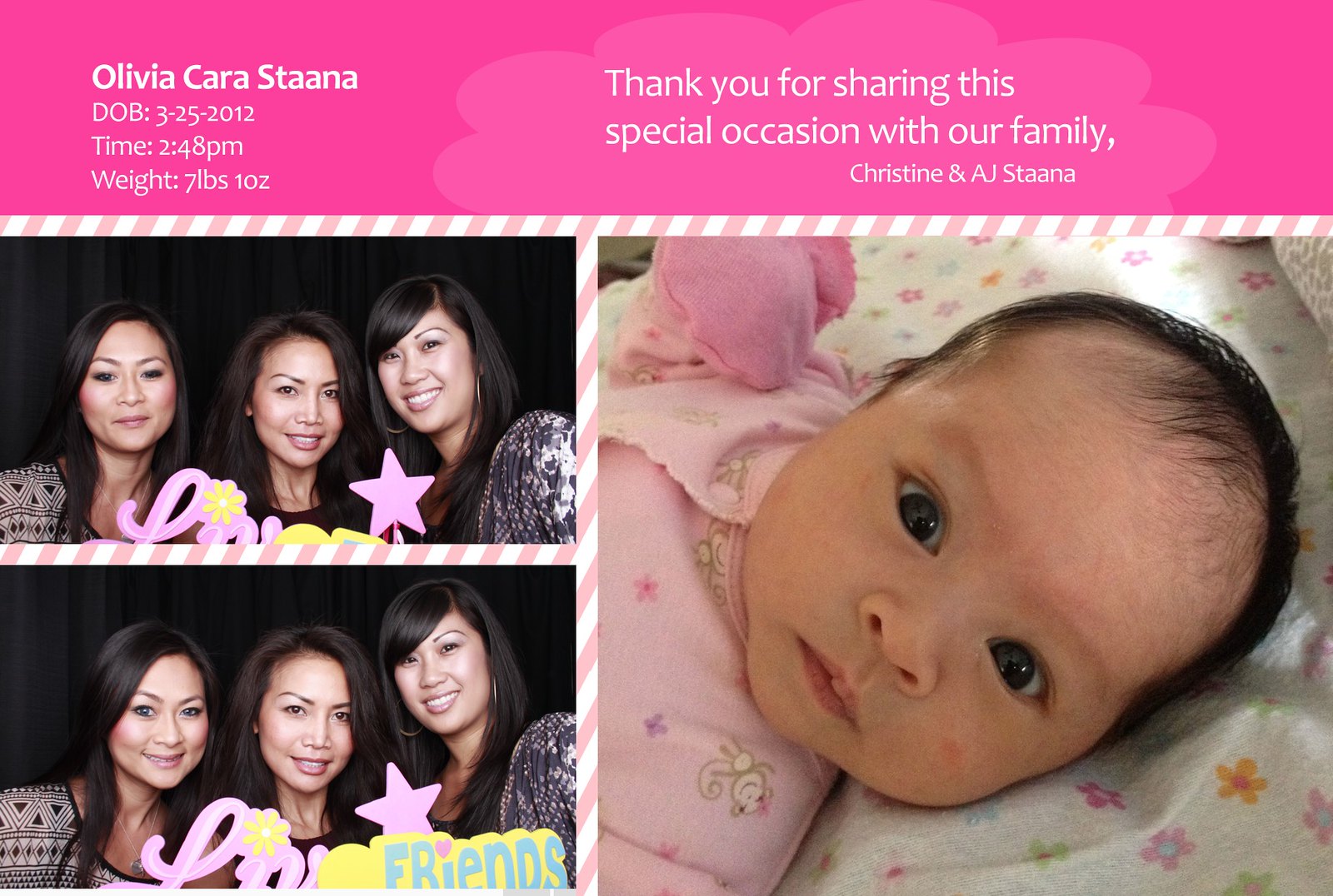This horizontal rectangular image is a detailed birth announcement with a prominent dark pink banner at the top. The banner features white left-aligned text that reads "Olivia Cara Stana," with the surname spelled out "S-T-A-A-N-A" in bold letters. Below, it lists her date of birth as "3-25-2012," the time "2:48 p.m.," and her weight "7 pounds 10 ounces." To the right within the pink area, it states, "Thank you for sharing this special occasion with our family," and is signed "Christine and A.J. Stana."

Beneath this heading, the image is divided into two main sections. On the right side, there's a large close-up photo of baby Olivia. She has short black hair and wide eyes, and is wearing a pink onesie with a monkey design. She is lying on a floral-patterned crib blanket, gazing directly at the camera with her mouth closed.

To the left of Olivia's photo, there are two smaller horizontal rectangular sections, each containing a picture of three women. The women all have long black hair and are looking at the camera, except for one who is glancing downward. They appear to be dressed in gray or black attire. The top photo has one woman holding a sign that reads, "friends" with a pink heart above the "i," while the bottom photo also includes some wording, although it is partially obscured. This celebratory announcement beautifully captures the joy and shared happiness of welcoming Olivia Cara Stana into the world.